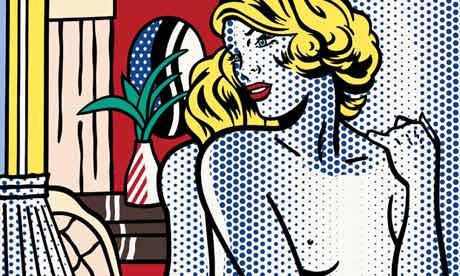The drawing is evocative of 1950s art characterized by an old-fashioned, comic-book style with a nod to Art Deco influences reminiscent of Andy Warhol. It showcases a topless woman with curly blonde hair and bright red lipstick, her body adorned with blue dots arranged in a dot matrix pattern that extends across the image, creating a sense of depth and shading. The woman is leaning against a mirror, which reflects the reverse image of her back and hair.

To her left, there's an old-fashioned white lampshade also covered in blue dots. Behind the woman, a beige curtain with yellow and white stripes can be seen on the left portion of the image. Further in the background, a brown table with white and red stripes holds a red and white striped vase filled with green, pointy leaves. The scene is set against a red wall decorated with blue dots or stars and black and white squiggles, adding to the vintage, whimsical atmosphere.